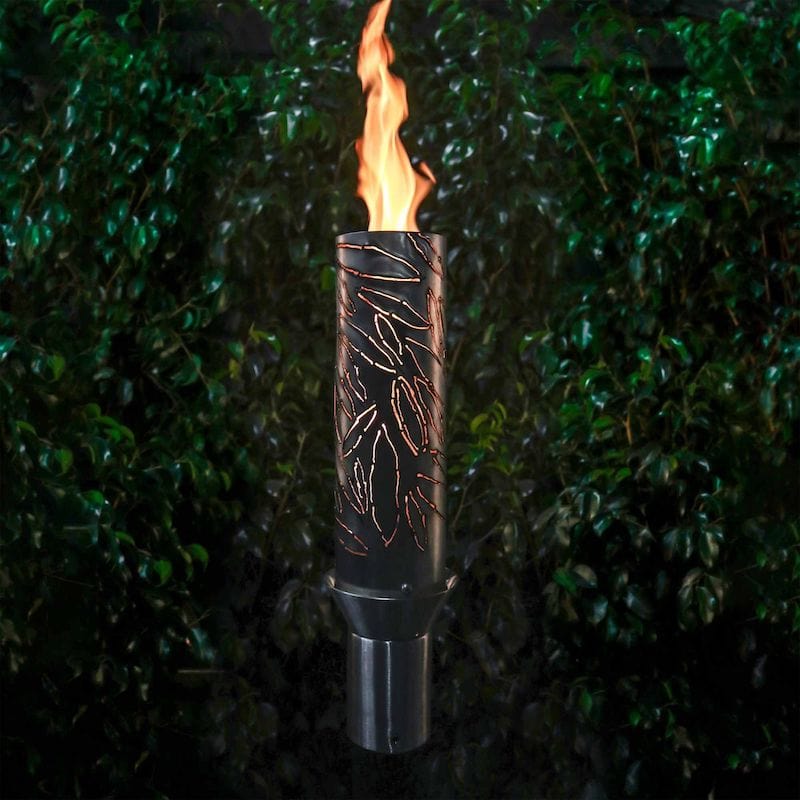The photograph showcases a tall, slender, metallic tiki torch with an intricate design featuring etched or cut-out leaf motifs. The torch stands against a densely textured backdrop of bright green foliage, presumably trees or bushes. The background is richly detailed, with leaves and twigs interspersed throughout, becoming less defined towards the darker bottom of the image. The flame emanating from the top of the torch is prominent, shooting up towards the upper third of the picture, and exhibits vivid hues of yellow and red. The glossy green leaves in the background reflect some of the torch's light, adding a dynamic interplay of light and shadow to the scene. The torch's base is black and shiny, transitioning to a brown section adorned with the etched leaf designs.